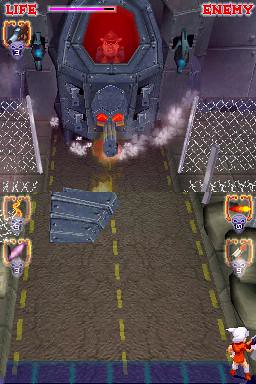This screenshot from a video game displays a detailed interface and environment. In the top-left corner, the word "Life" is prominently displayed, while the top-right corner features the word "Enemy" in bold red block letters outlined in white. At the center top of the image, a gray structure is visible, topped with a red hexagonal shape, possibly indicating a light or signal. The majority of the image is dominated by an asphalt road, marked by a dotted yellow line in the center and additional dotted yellow lines on either side. Midway along the left and right edges of the image, chain-link fences are discernible. In the lower right-hand corner, one of the game's characters is visible, seemingly a soldier dressed in a white helmet and a red and white uniform.